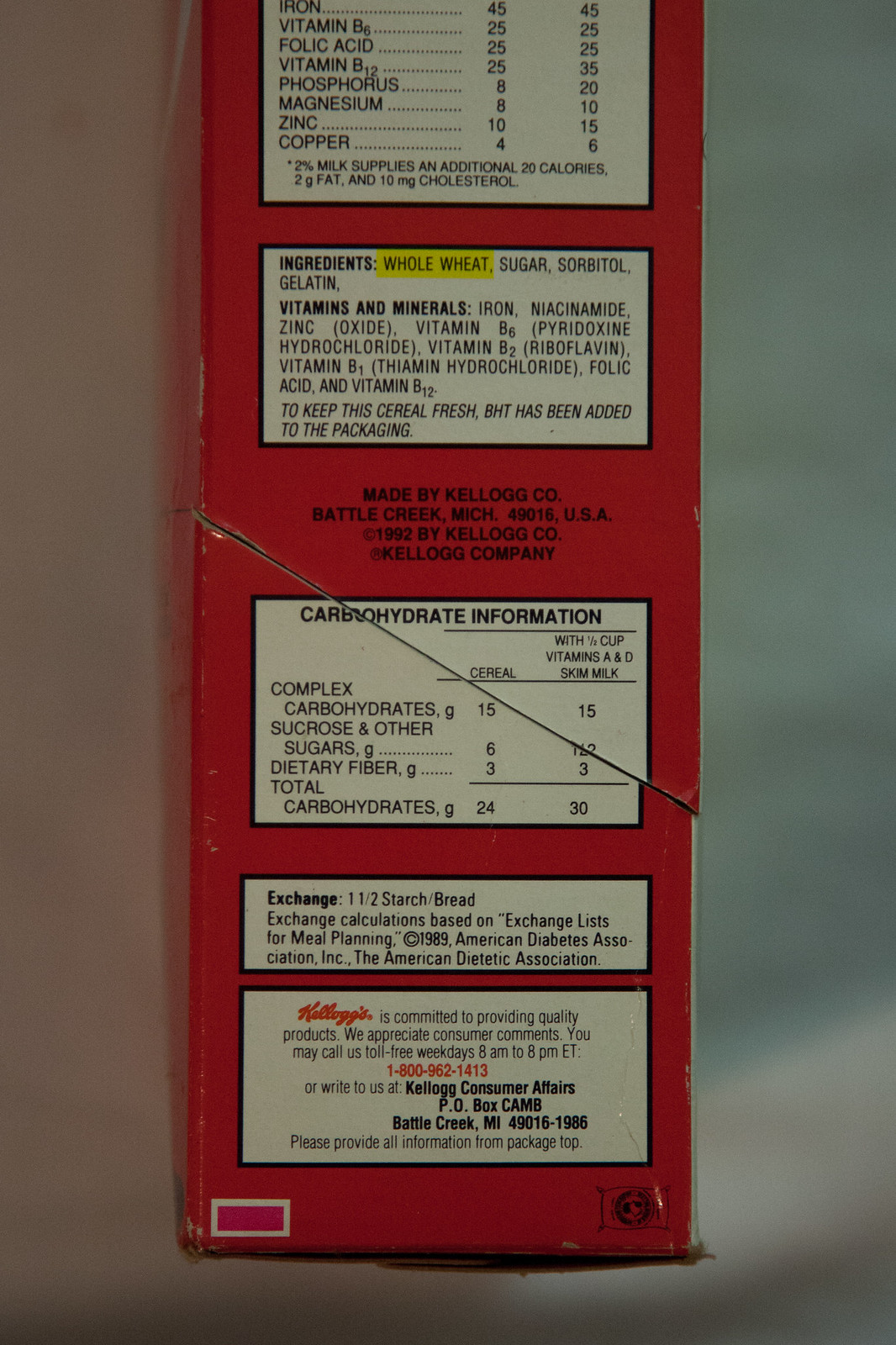The photograph depicts the side of a red box, likely containing a food item. Prominently displayed on the side are white square labels, which include a partially visible nutrition information chart and a list of ingredients. The label indicates that the food item is produced by Kellogg Co., USA, based in Battle Creek, Michigan, renowned for its cereal products. The ingredients listed include whole wheat, sugar, sorbitol, and gelatin, suggesting it may be a type of cereal, though the exact product cannot be determined from this partial view. Additionally, some information about the vitamins and minerals present in the product is visible, but the full details are obscured.